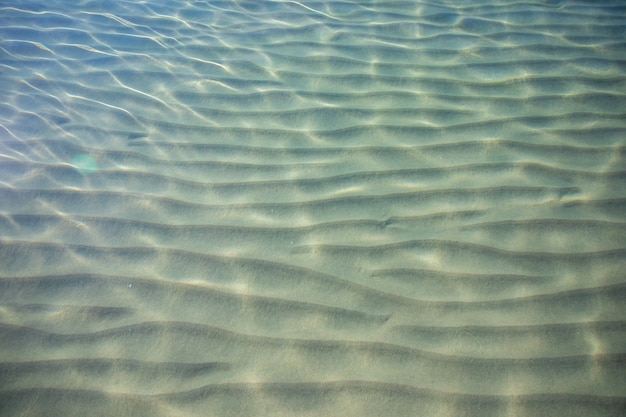This underwater photo captures a vibrant and sunlit scene of a sandy seafloor. The clear water reveals the sandy bottom, which is rippled with wavy ridges stretching horizontally from the left to the right. The ripples become tighter in the distance toward the top of the square-shaped image. Sunlight penetrates the water's surface, creating refracted light patterns and white veins across the yellow-tan sand, enhancing the natural beauty of the scene. On the left side of the image, a round teal dot adds an additional point of interest. Overall, the bright and clear environment underscores the serene and natural underwater setting.